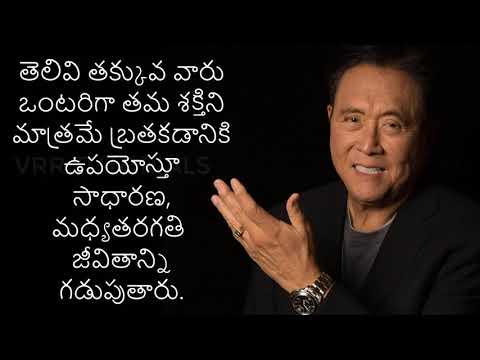The image features a middle-aged Asian man with dark hair and a clean-shaven face, who is in the midst of explaining or discussing something, with his mouth open and teeth visible in what appears to be mid-speech. He is dressed in a black blazer over a gray shirt and sports a silver watch on his left wrist, indicating a time around 3:45 or 4:45, along with a gold ring on the ring finger of the same hand. The man is gesturing towards text in a foreign language, possibly Arabic, displayed to the left side of the image. This text consists of eight lines in a white font against a dark gray or black background. The main colors in the photo are black, gray, and white. He appears to be addressing the camera directly, creating an impression of either teaching or explaining something to an audience.